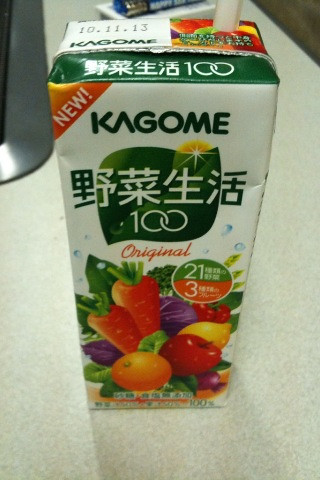This is a portrait-style image of a rectangular juice box labeled "Kagome," captured in sharp focus while standing on a white, formica-like surface. The background of the photo is blurred, directing full attention to the juice box at the center. The top of the box features a date, "10.11.13," situated above the brand name "Kagome" written in green. A straw has been inserted into the top-right corner of the box. 

Beneath the brand name, there's an orange text labeled "Original," and it includes numbers "100" and additional text in Japanese, suggesting it's an Asian-style juice. The top-left corner of the carton features a "New!" label in white, set against an orange triangle.

The bottom section of the juice box illustrates a vibrant array of fruits and vegetables, including carrots, bell peppers, onions, lemons, oranges, red apples, green vegetables, and some purple produce. The side of the box also highlights "21" in green and "3" in orange, suggesting nutritional information or ingredient quantities. A small silver object can be seen in the top-left corner of the white platform surface.